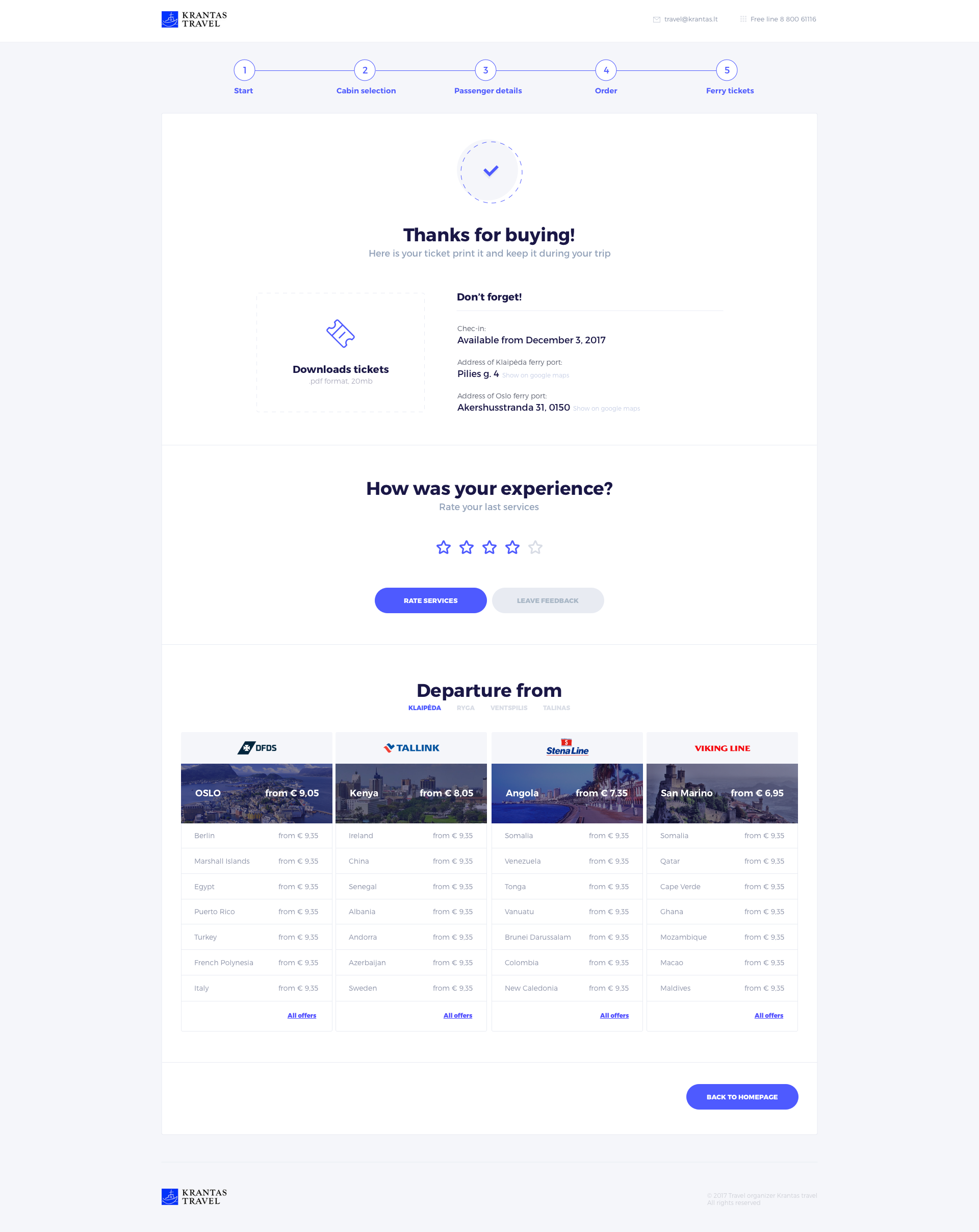The image is a small, blurry screenshot of a website page, which appears to be named "Cranton Travel". Despite the small size, several elements on the webpage are distinguishable. The top section prominently displays the text "Thanks for buying" in bold, followed by a large heading in the middle that reads "How was your experience?" Below these, there is a sequence of labels indicating a multi-step process, starting with "Step 1: Start", followed by steps 2 through 5, although the exact details of steps 2 through 5 are unclear. 

A check mark icon below the step sequence reiterates "Thanks for buying". To the left of this, there's an option to "Download tickets", while to the right, a section titled "Don't forget" provides reminders related to the flight. Under the "How was your experience?" heading, there is a star rating system, with four clickable blue stars and a fifth star that appears inactive or unselectable.

Further down are two unreadable buttons, potentially for submitting feedback. The last section addressed is titled "Departure from", featuring four small images presumably related to different flights, followed by rows and columns that likely contain detailed flight information. The primary colors of the webpage include dark periwinkle, cobalt blue, black, white, gray, cream, red, and green.